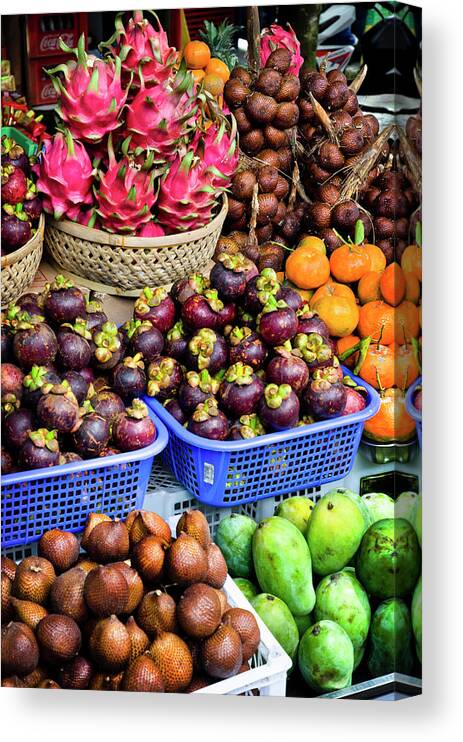This photorealistic image captures an outdoor fruit stand, likely set in a tropical market scenario, abundant with vibrantly colored fruits organized meticulously in various containers. On the lowest layer nearest to the bottom of the image, peculiar brown, round, and textured fruits are showcased in a white bin on the left and adjacent to it on the right, larger oblong green melons are displayed. Elevating to the next layer, two small blue containers brim with small, round, purple fruits adorned with green stems. To the right of these, smaller, round, orange fruits offer a contrast. Above, a wicker basket extends off the left edge containing fruits similar to those in the second layer. Another wicker basket on the same higher level houses an eye-catching collection of pink and green dragon fruits stacked meticulously. To the right, more brown and interestingly textured fruits, akin to the ones on the layer below, continue the display. In the background, partially obscured but noticeable in the top left corner, are vibrant red crates of Coca-Cola drinks, adding a familiar element to the exotic assortment of produce. The fruits and vegetables, along with the arrangement in white bins, blue plastic baskets, and wicker baskets, depict a rich and diverse market atmosphere often found in tropical locales.